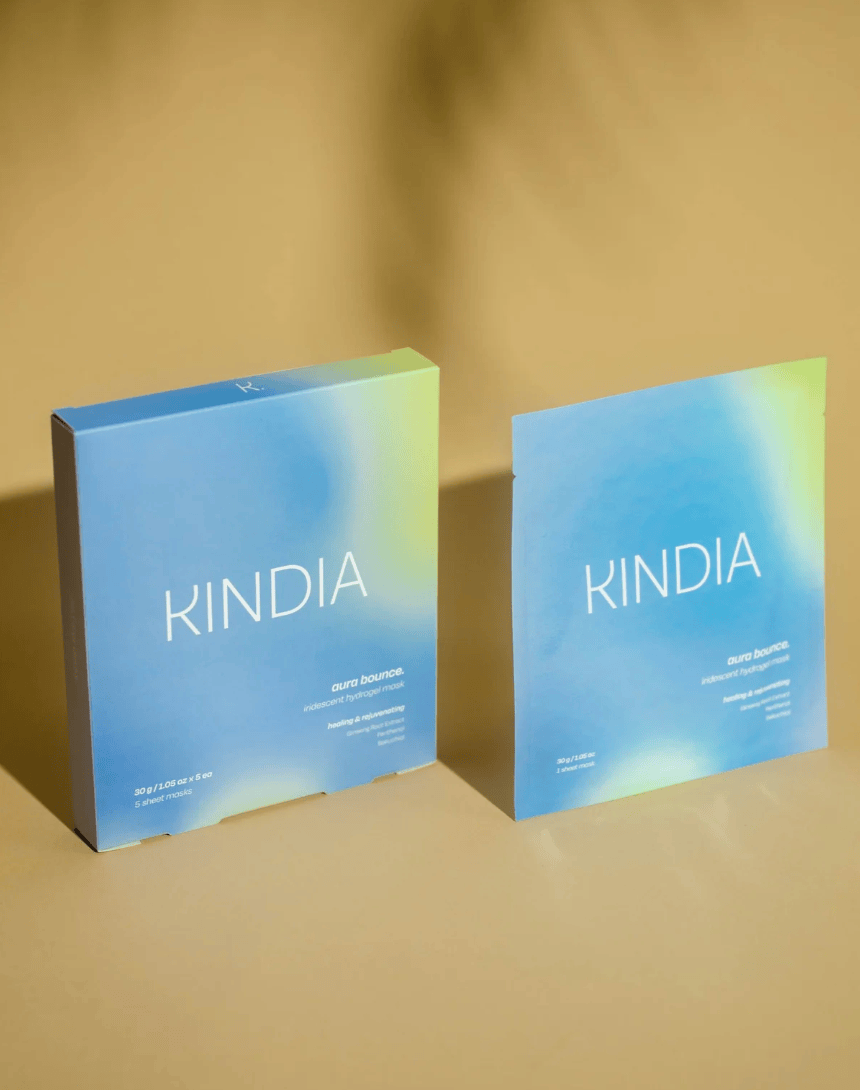In a product presentation photo, two items from the brand "Kindia" are prominently displayed against a beige background. Both items, a product box on the left and a single, individually packaged sheet mask on the right, feature blue packaging with light green and white accents. The text "Kindia" is stylized in a white font, though additional small white writing details are difficult to discern. The larger box likely contains five sheet masks, while the packet holds one. The packaging reads "Kindia Incandescent Hydrogel Mask Healing and Rejuvenating, 30 grams." A shadow, possibly from a nearby plant, is cast across the scene, accentuating the direct light illuminating the setup. The items stand on a yellowish surface, with a clear indication of a rip-top opening on the single mask packet.